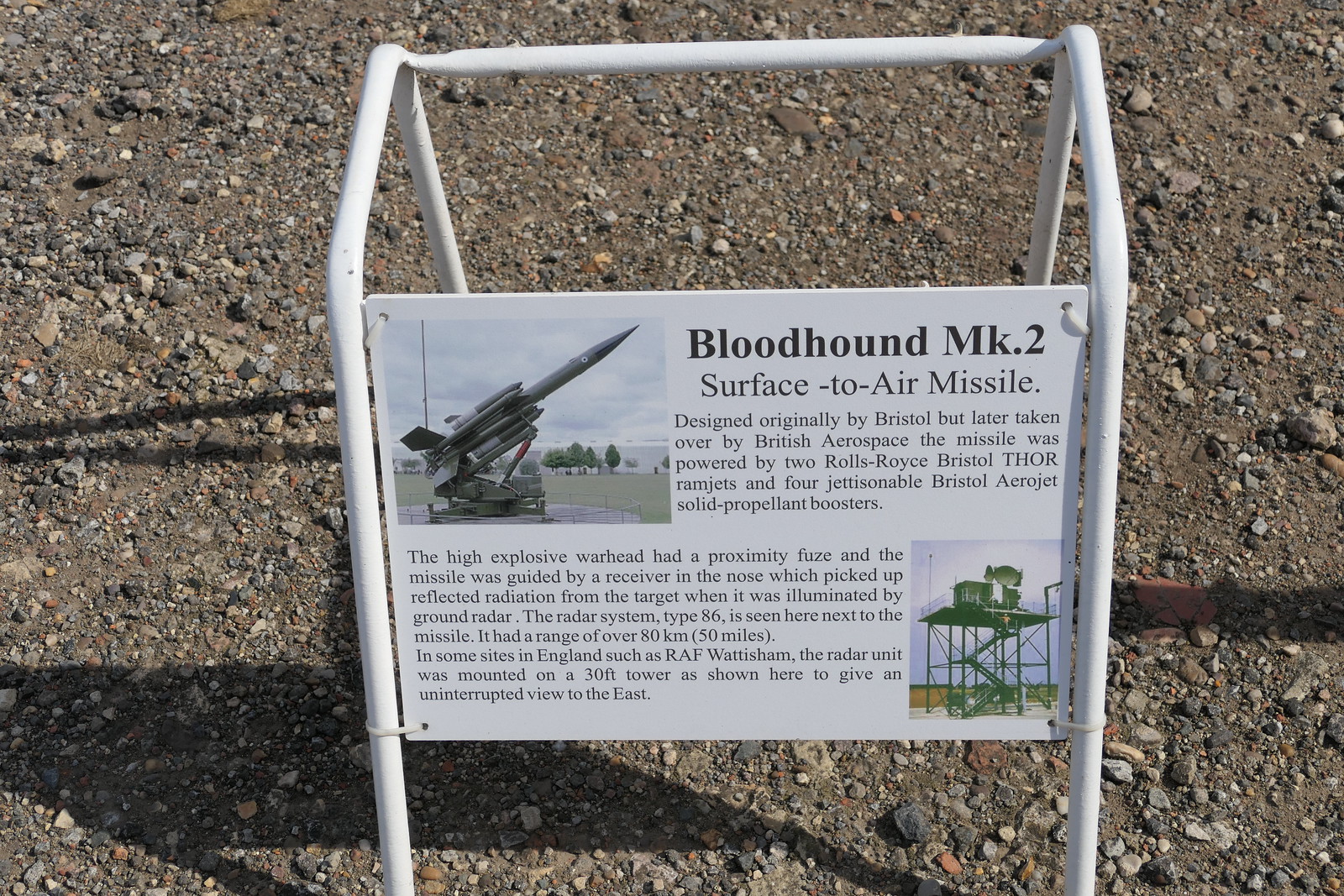The photograph captures an outdoor scene during daylight, featuring a white metal stand with four legs positioned on a brown, rocky patch of soil scattered with variously shaped and colored pebbles. Mounted on the stand is a white informational sign that clearly exhibits two images: one in the top left corner illustrating what appears to be a rocket or missile, and another in the bottom right corner showing a structure built on an iron framework along with some radar antennae and a building atop the structure. 

The sign is detailed and reads: "Bloodhound Mk2 Surface-to-Air Missile, originally designed by Bristol but later managed by British Aerospace. The missile was propelled by two Rolls-Royce Bristol Thor ramjets and equipped with four jettisonable Bristol Aerojet solid propellant boosters. It utilized a high explosive warhead with a proximity fuse and was guided by a receiver in the nose, which picked up reflected radiation from the target when illuminated by ground radar." The sign further elaborates on the radar system: "The radar system Type 86, depicted next to the missile, had a range exceeding 80 kilometers (50 miles). At specific sites in England, such as RAF Waddesham, the radar unit was mounted on a 30-foot tower, as shown here, to ensure an uninterrupted view to the east."

The image associated with the missile includes background elements like trees, while the structure on the right-hand side features stairs leading up to the tower, contributing to the detailed context of the display.